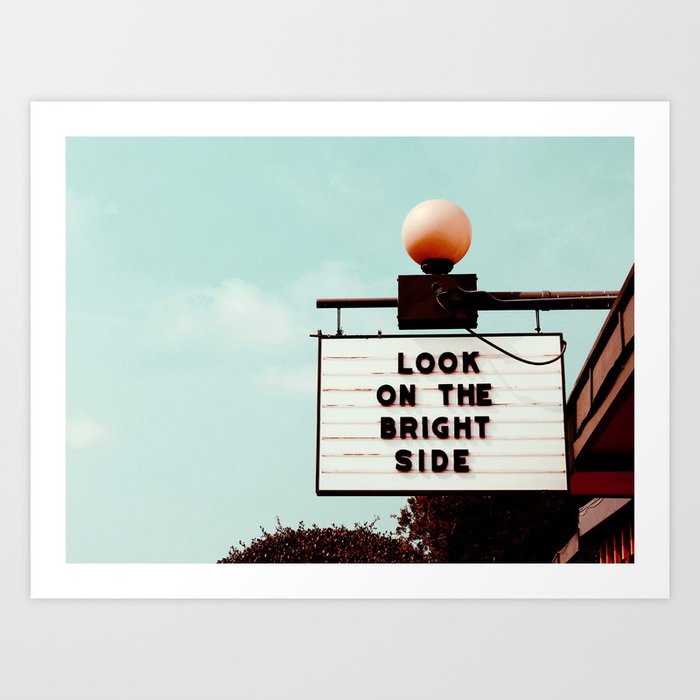In this vibrant outdoor scene, a prominent sign stands out against a pale blue, cloud-dappled sky. The sign, mounted on a building, displays the optimistic message "LOOK ON THE BRIGHT SIDE" in bold black capital letters set against a white background. This classic style sign, reminiscent of old-school marquee boards, is meticulously arranged with each letter manually positioned. Above the sign, a unique peach-colored, globe-shaped lamp is affixed, casting light to emphasize the message, with its supporting wire and metal bracket clearly visible. The lower right corner of the image reveals a snippet of a building adorned with a touch of red, providing a contrasting splash of color. To the side, the presence of trees adds a hint of natural serenity to the urban scene. The composition is framed within a horizontal, rectangular white border, capturing a serene and motivational snapshot that merges natural and man-made elements seamlessly.